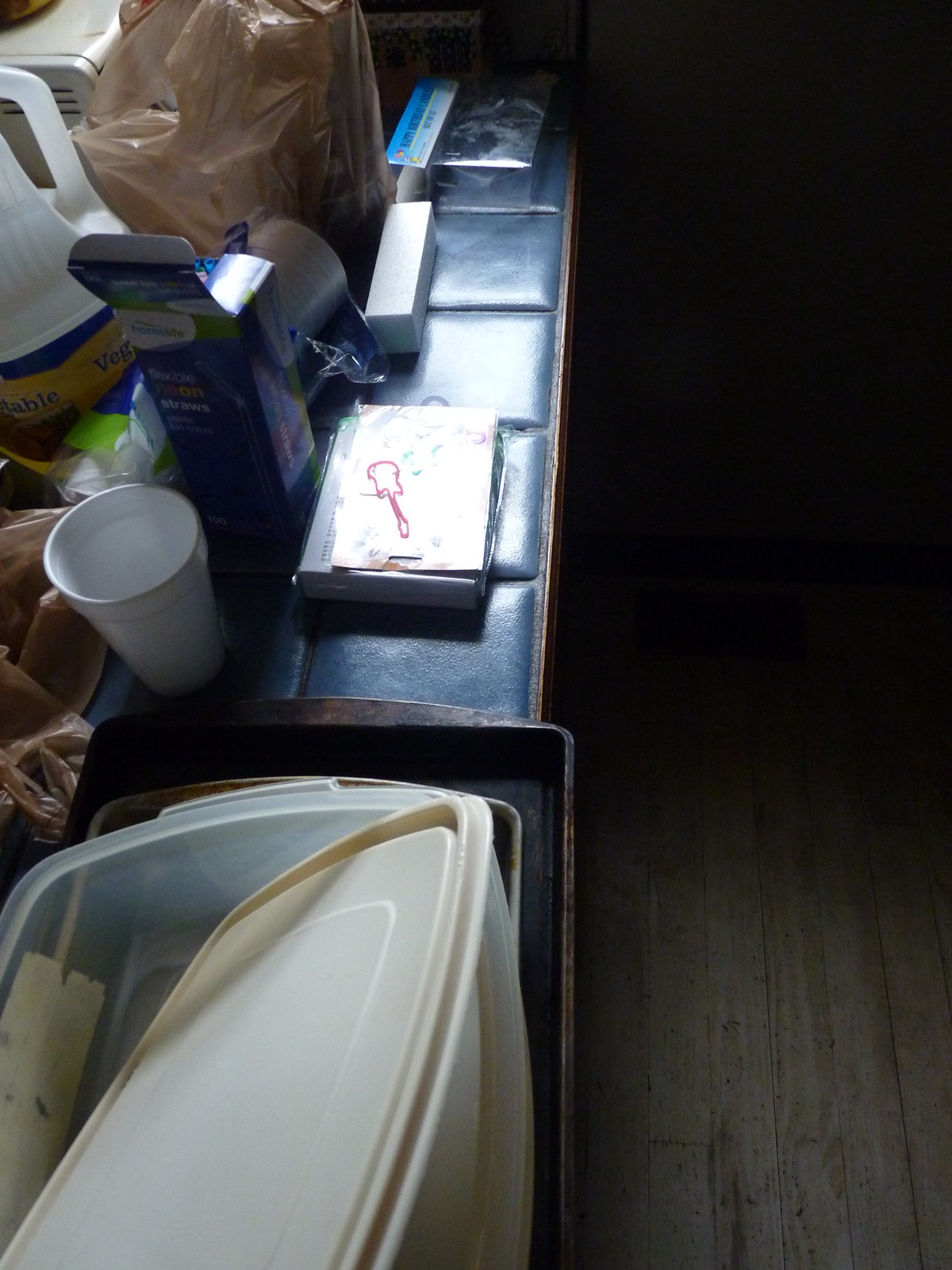The image showcases a section of a home, potentially part of a living room or a kitchen counter. The area is cluttered with various household items. Dominating the countertop, which consists of blue square tiles, is a large jug labeled "Vegetable," likely containing vegetable oil. Nearby, an open box labeled "Flexible Neon Straws" sits among other indistinguishable boxes, one of which is adorned with a guitar-shaped silly band, reflecting light and obscuring further details. Additionally, a package of Styrofoam cups and several grocery bags, their contents concealed, are scattered across the space. In the lower portion of the image, a pan is visible, holding a dish and a plastic bowl, the lid resting inside. To the right, the wooden floor transitions from the countertop area, adding a warm contrast to the scene.